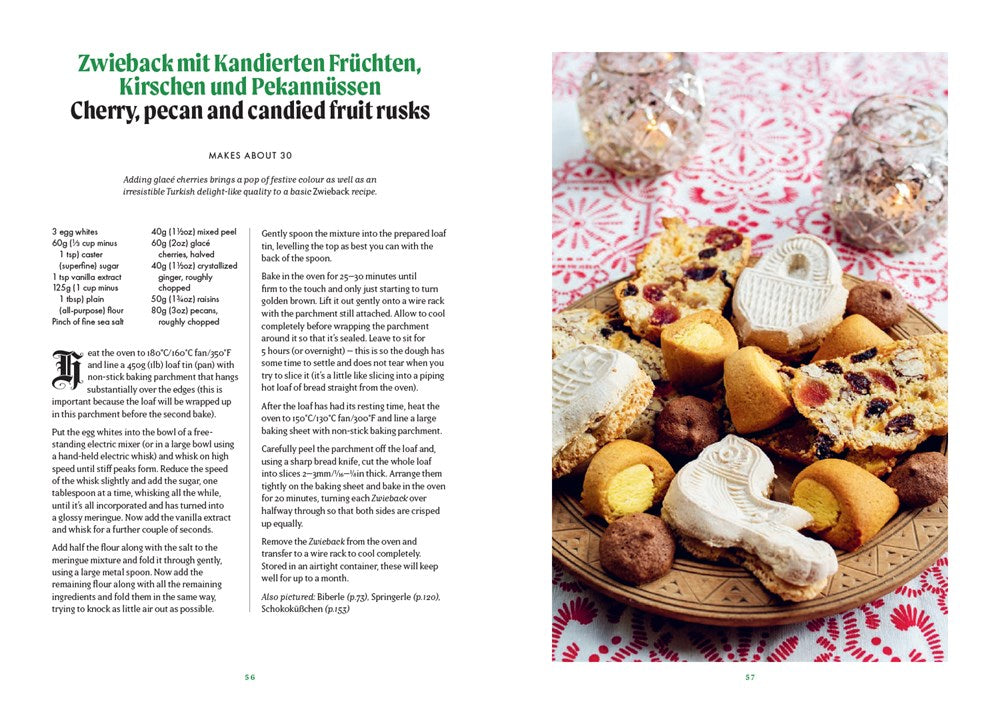The image captures an open page of a cooking magazine. On the left side, the title of the recipe is written in German and then translated to English as "Cherry, Pecan, and Candied Fruit Rusks." The recipe, which makes about 30 treats, describes a process that begins with three egg whites and mentions adding cherries for a pop of festive color and a light, Turkish delight-like quality. On the right side of the page, a beautifully arranged wooden circular plate sits on a white surface with red flower patterns, resembling doilies. The plate holds an assortment of cookies and desserts, including white and brown rose-shaped treats, circular candies, and pieces resembling fruit cake and raisin bread. In the background, two lit glass candles with delicate flames add a warm, inviting atmosphere to the scene.